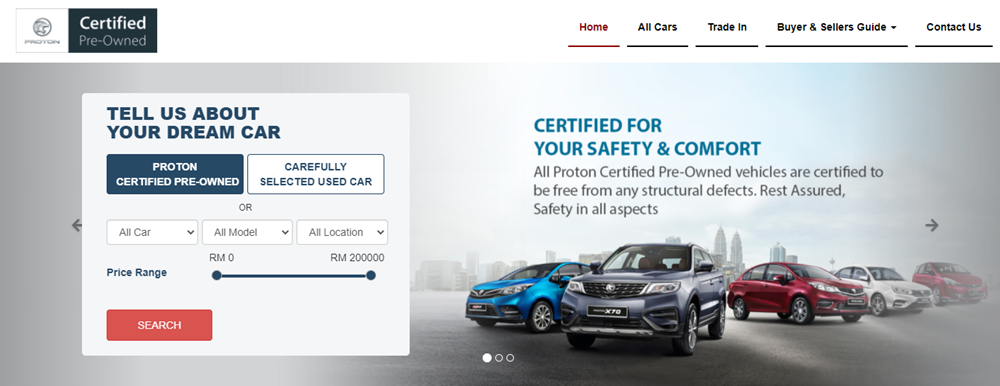**Website Caption for Proton Certified Pre-Owned Cars**

Welcome to our Proton Certified Pre-Owned car dealership's website. At the top navigation bar, you'll find easy access to various sections: Home, All Cars, Trade-In, Buyer's and Seller's Guide, and Contact Us.

**Filter and Search Options:**
On the left side of the page, there's a gray square offering a prompt in blue letters: "Tell us about your dream car." Below that, you'll discover a blue box with white letters proclaiming "Proton Certified Pre-Owned." Underneath is a white box with blue letters stating "Carefully Selected Used Cars." 

Here, you can filter and select vehicles based on various criteria, including make, model, location, and price range. There's also a user-friendly drop-down menu and a prominent search button to help streamline your vehicle search.

**Vehicle Display:**
The main section features a dynamic image set against a gray background with a cityscape. In the foreground, a variety of certified pre-owned vehicles are showcased, including a blue coupe, a gray SUV, a red sedan, a white sedan, and another compact red car. Our selection is diverse, catering to different preferences and needs, ensuring you find the perfect car.

Explore our extensive range and discover your ideal certified pre-owned vehicle today with confidence at Proton.